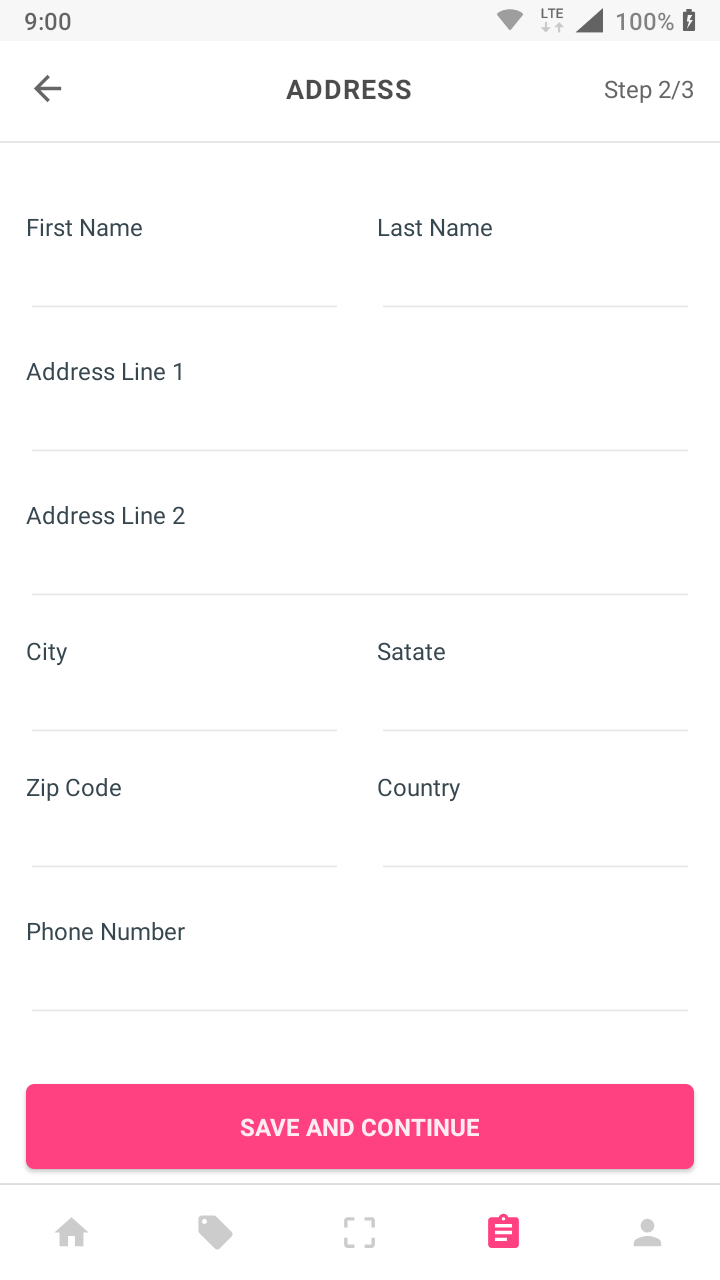The image is a screenshot from a mobile phone, displaying a form interface on a clean, white background. At the top of the screen, there is a gray bar displaying essential status icons: the time reads 9:00, the phone indicates an LTE connection, and the battery is fully charged at 100%. Below this bar, an arrow pointing left and the word "address" is visible, denoting navigation or progress. The form is identified as "Step 2 out of 3."

The form fields are arranged vertically, prompting the user to input their personal information: first name, last name, address line 1, address line 2, city, state, zip code (on the left), country (on the right), and phone number. At the bottom of the form, there's a prominent, reddish-pink button with the text "SAVE AND CONTINUE" in bold, white, capital letters.

At the very bottom of the screen, there is a navigation bar featuring five icons: a house, a ticket, a square, a notepad, and a silhouette of a human, likely representing different sections or features of the app.